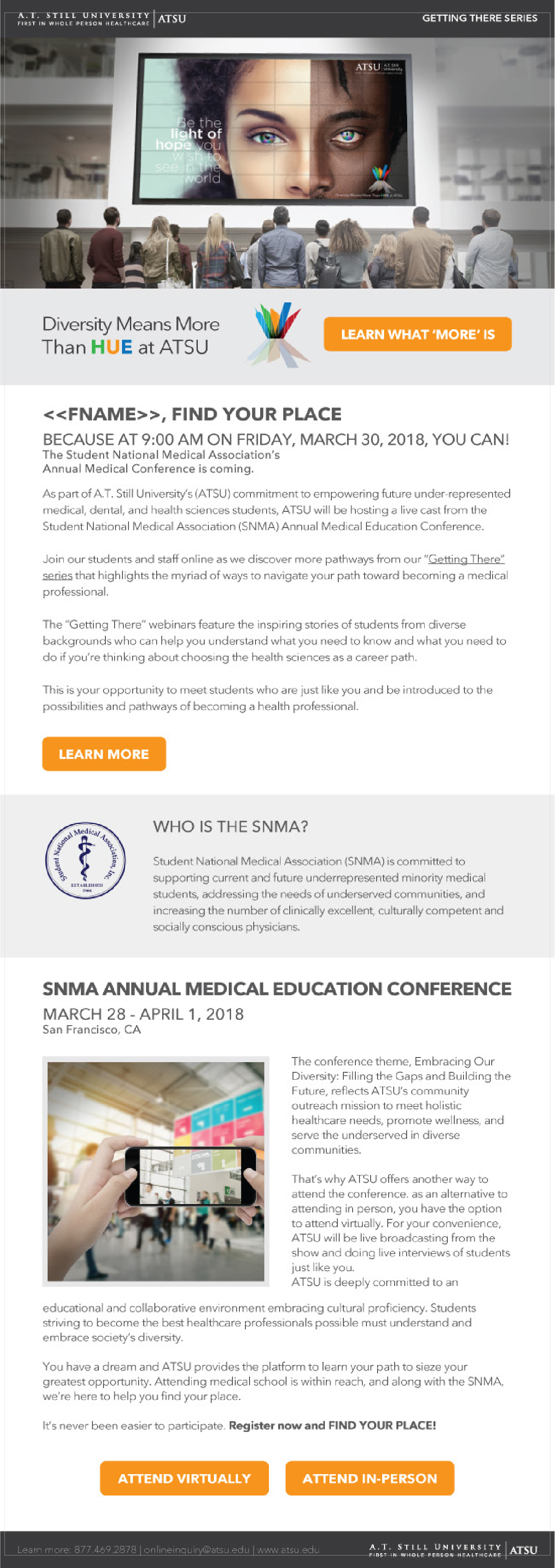The image is a screen grab of a website. At the top, the website’s title or menu bar is somewhat blurry and difficult to read. Below this bar, the main image depicts a group of people looking up at a large screen. The screen prominently features a woman’s face, with half of her face having light skin, blue eyes, and curly hair, and the other half having dark skin and black hair, symbolizing diversity.

Overlaid on this image is the text, "Diversity means more than H-U-E at ATSU." The letters "H," "U," and "E" are color-coded as green, orange, and blue, respectively. Beneath this text, there is a colorful logo followed by the phrases "Learn what more is" and "Find your place."

Further down, details about an upcoming event are provided: "Friday, March 30, 2018, at 9 AM, the Student National Medical Association's Annual Medical Conference." Some smaller, blurry text follows, which is difficult to read, and there is a "Learn More" button.

Directly below that section, there is a gray area with a circular logo and the heading "Who is the SNMA?" An explanatory text follows, in smaller font. Prominently displayed in bold text is "SNMA Annual Medical Education Conference," with additional details: "March 28 through April 1, 2018, San Francisco, CA." It also mentions that attendees can "Attend virtually and in person."